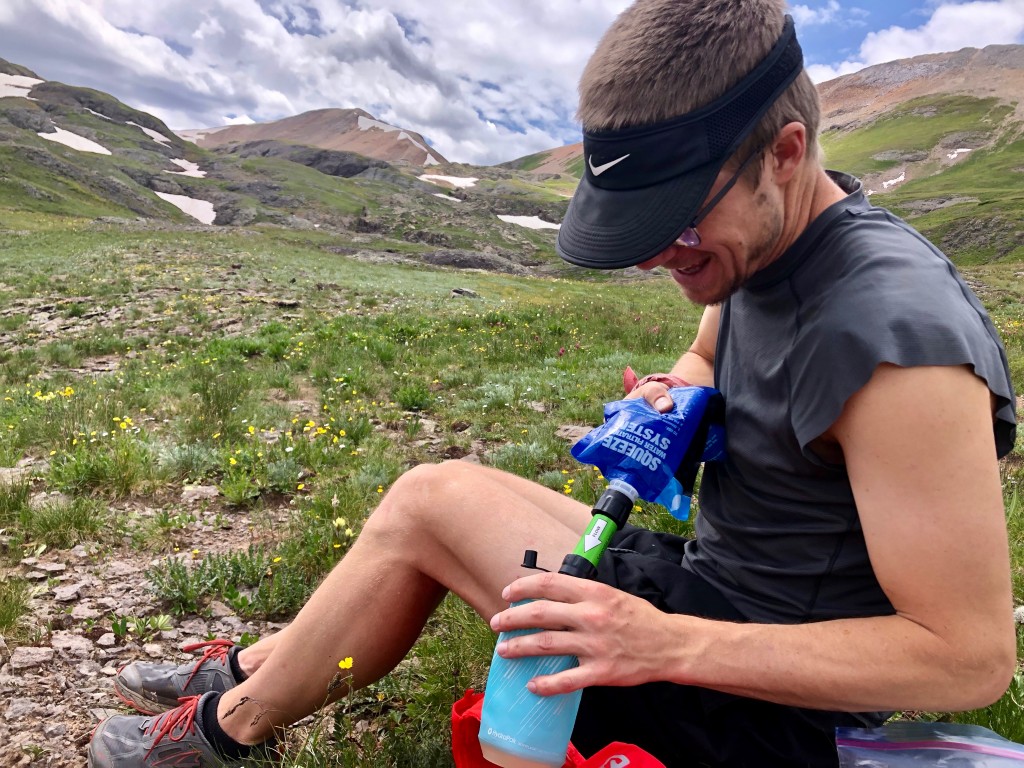Photograph of a man of European descent sitting on the grass in a bright mountain valley. He is surrounded by lush grass and a few yellow flowers, under cloudy but somewhat blue skies. In the background, small, mostly brown and gray mountain peaks are visible, some with patches of snow. The man, who has short dark hair, is wearing a gray Nike sun visor, prescription glasses, a gray cut-off t-shirt, black shorts, black ankle socks, and gray hiking sneakers with red laces. He is smiling and looking down as he squeezes a blue hydration drink from a container labeled "squeeze" into a plastic water bottle, using a green connector. An orange item, possibly a jacket, is partially visible underneath the bottle, and a plastic Ziploc bag is directly behind him. There are no trees and no other people around.